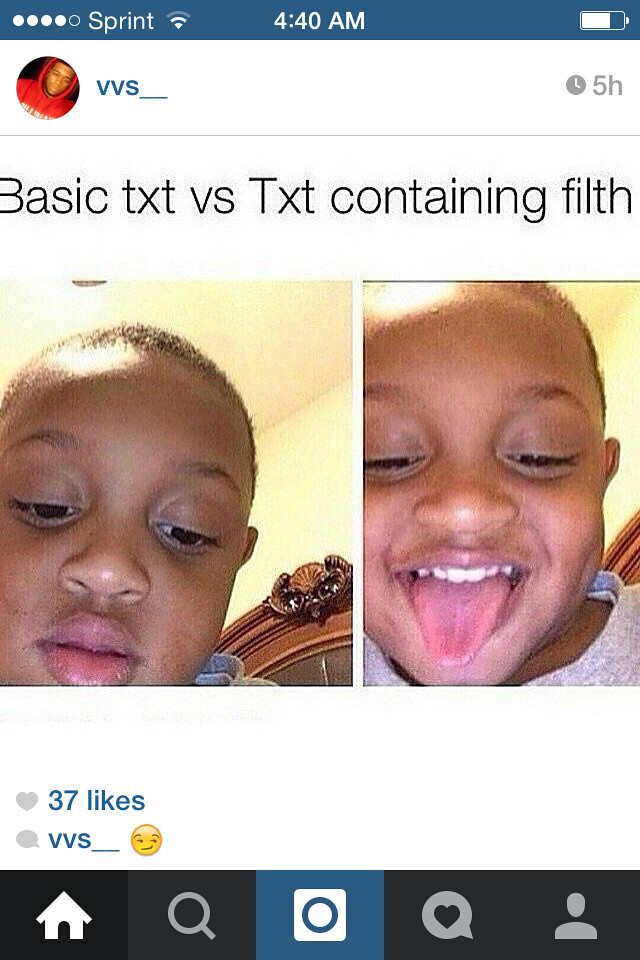This image is a screenshot of a social media meme viewed on a cell phone. At the top left of the screen, there is a blue bar displaying four out of five signal strength bars, indicating the provider is Sprint. The time is shown in the center as 4:40 a.m., and the battery icon on the top right shows approximately two-thirds remaining power.

Below this, there is a red circular profile picture of a man wearing a red hoodie, labeled with the username "vvs__," followed by a time clock symbol indicating the post was made 5 hours ago. The meme caption reads "Basic TXT versus TXT containing filth" and features two side-by-side images of a young black boy. In the left image, the boy looks downwards against a yellow ceiling and wall, next to a mirror with a wooden frame. In the right image, the boy is sticking out his tongue and smiling. At the bottom of the meme, there is a heart icon with a count of 37 likes displayed.